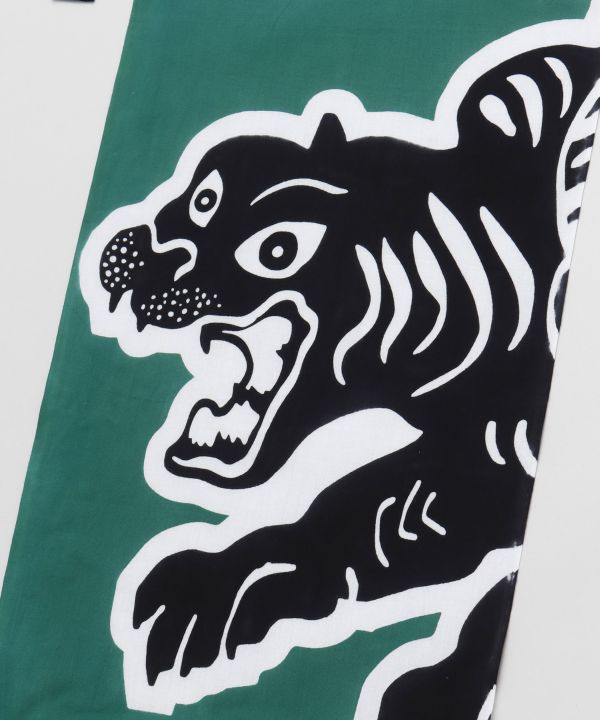This is an image depicting a fierce-looking black and white tiger, possibly designed in a traditional tattoo style. The tiger is shown with its mouth wide open, displaying sharp black teeth and white pupils within large, angled eyes that enhance its vicious expression. The image is set diagonally on a forest green background, bordered by a white outline. The tiger's body is only partially visible, extending from the shoulders to its head, with one paw extended in an attack stance. Its stripes are white against the predominantly black body, highlighted to accentuate its ferocity. The overall presentation suggests it could be printed on a piece of cloth or a flag, perhaps for a sports team, although the material is not distinctly identifiable beyond the greenish-blue backdrop.